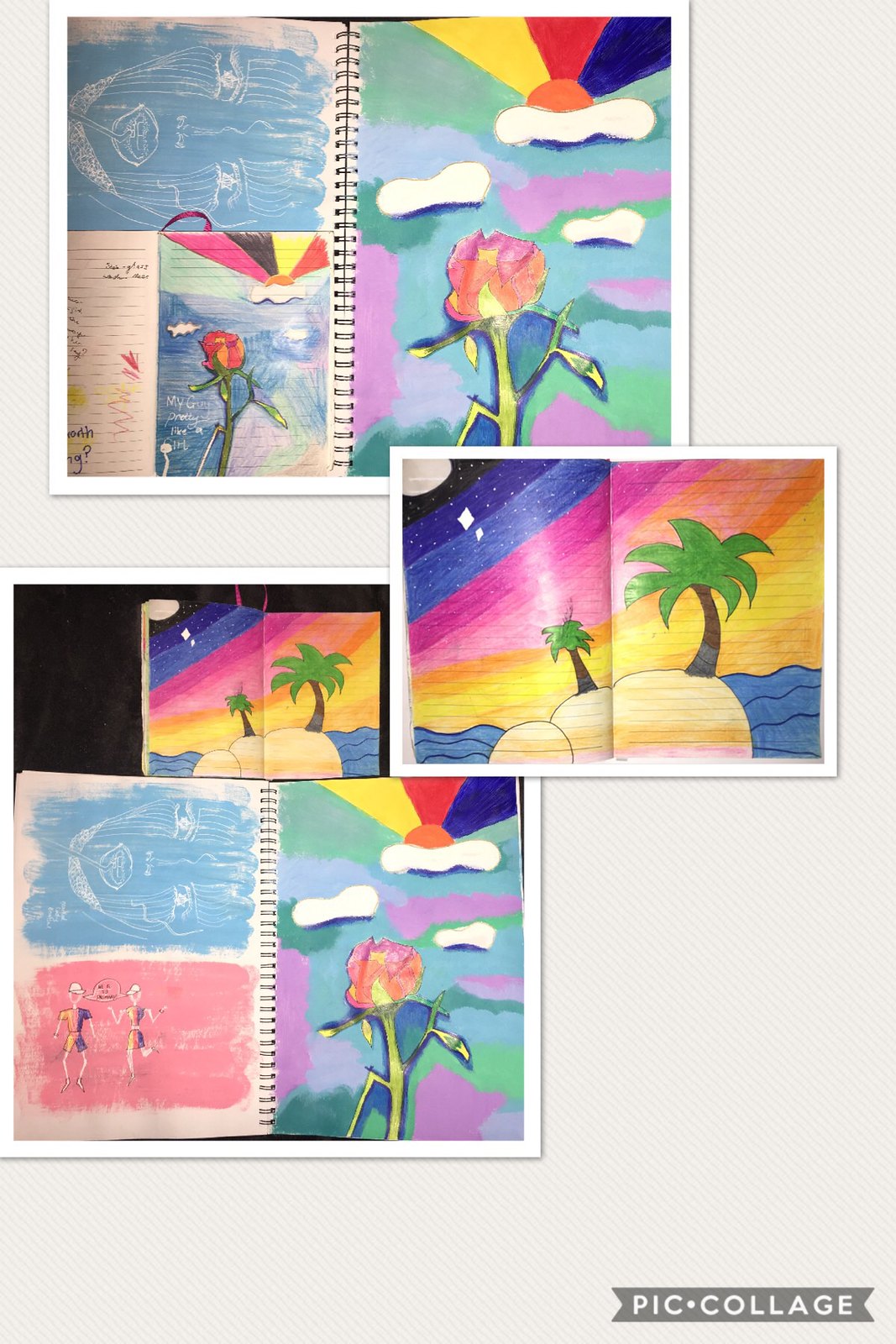In this rectangular image, there are three distinct areas showcasing various artworks. At the top, an open sketchbook is displayed, revealing a vibrant collection of hand-drawn illustrations. One of the notable sketches depicts a whimsical flower with a pink blossom that transitions into dancing legs, imitating roots. Adjacent to it, in the upper right corner of the sketchbook, the bottom of a hot air balloon can be seen, presented in primary colors of yellow, red, and blue, floating above a small cloud.

Beneath the sketchbook, the second artwork features an idyllic island scene. A tall palm tree stands prominently amidst a colorful landscape, seemingly created with crayon, with the background displaying a wavy ocean that adds to the serene atmosphere.

In the lower left corner of the image, there are areas filled with pink and pale blue hues. Among these colors, there are scribbled, almost ethereal depictions of a human face drawn in white, showing a sideways profile with the mouth on the left and two eyes aligned vertically.